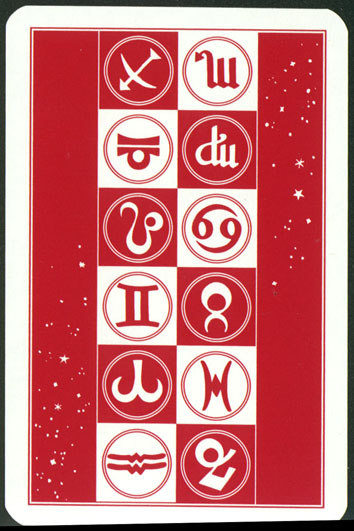This image showcases an intricate design on a white background bordered by a black frame. The primary canvas of the image is a vivid red. Adorning each border are small white stars, emerging from the left corners and descending from the right corners, creating a dynamic visual effect. Central to the composition are two perfectly aligned vertical columns of enigmatic symbols, divided into six rows. These rows alternate between a red background with a white symbol encased in a white circle and a white background with a red symbol encased in a red circle. The symbols themselves are mysterious and do not resemble any known alphabet or modern iconography. Instead, they appear purely decorative, featuring a variety of intricate lines and swirling patterns, some intersecting while others run parallel. The overall effect is one of ceremonial elegance and cryptic beauty.